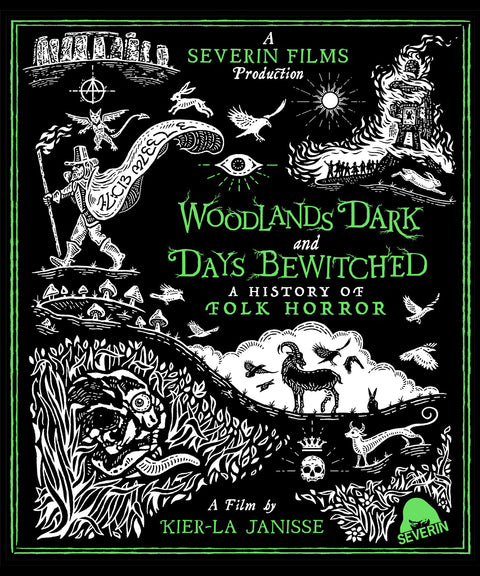The image is a movie poster with a predominantly black background, adorned with intricate white and electric green illustrations, creating a striking contrast. The textured effect suggests the appearance of white paint on a scraped black surface, revealing the underlying white. This poster advertises "Woodlands Dark and Days Bewitched: A History of Folk Horror," a Severin Films production directed by Keir La Janisse. The imagery evokes a haunting, witchcraft-related theme, featuring a variety of spooky elements: a flying devil in the upper left, a colonist-hatted man possibly representing a warlock, an all-seeing eye, rabbits, eagles or hawks, a Capricorn-like goat with ominous clouds, sinister birds, mushrooms, and a crowned skull. Additionally, there's a critter in the bottom left that resembles a dragon standing in water. The landscape also includes a wheat field, a moon, and what might be a castle or a gathering of people ascending a hill, contributing to the eerie, folk horror ambiance.